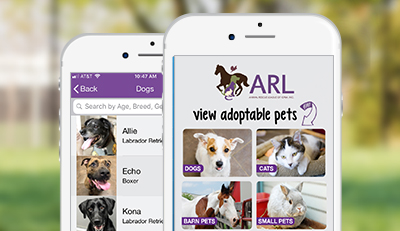The image appears to be an online advertisement for pet adoption, featuring two overlapping silver and white cell phones. The phone on the right partially obscures the one on the left. 

The screen of the phone on the right displays an app from "ARL" (presumably the Animal Rescue League), with the title in purple at the top followed by "View Adoptable Pets" in black. Four sections categorized by pet types are visible. The upper left section features a white and brown dog under "Dogs." The upper right section shows a black cat looking at the camera under "Cats." The bottom left section displays a white and brown horse and is labeled "Barn Pets." Lastly, the bottom right section showcases a gray bunny under "Small Pets."

The phone on the left highlights more detailed information. At the top, a search bar is visible, with "Dogs" selected. Below the search bar, three pets are listed with their images and descriptions. The first is a black dog named "Allie," categorized as a Labrador. The second is a brown and black dog named "Echo," identified as a Boxer. The third is a black dog named "Kona," labeled as a Labrador Retriever. 

The background of the image is blurred, indicating an outdoor setting with green trees and grass, softly illuminated by natural light.